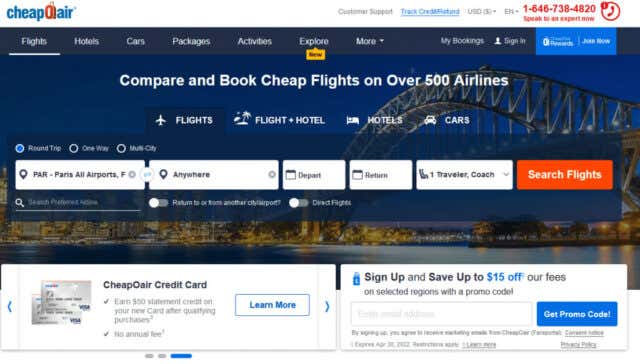This detailed image captures the user interface of the "Cheap Air" website. The brand name "Cheap Air" is prominently displayed at the top, with "Cheap" in blue font and "Air" also in blue font, separated by a distinctive symbol resembling a large "O" in a reddish color. 

In the upper right-hand corner of the image, there's a clearly visible telephone number, facilitating direct customer support. Below the contact number, a horizontal menu bar is located, presenting various navigation options such as "Flights," "Hotels," "Cars," "Packages," "Activities," "Explore," and "More."

The central part of the webpage showcases a bold, white text banner with a compelling call to action: "Compare and book Cheap flights on over 500 airlines." Directly underneath this banner, in a smaller font, are selectable tabs labeled "Flights," "Flights and Hotels," and "Cars."

Further down the page, users can see an input section for conducting searches. This section provides multiple search options, presumably five, allowing users to input criteria for their desired flights. The available search categories include options like "Deposit," "Returns," and "Traveler's Coach."

The layout and design elements are clearly structured to assist users in navigating the site efficiently and booking their travel plans with ease.